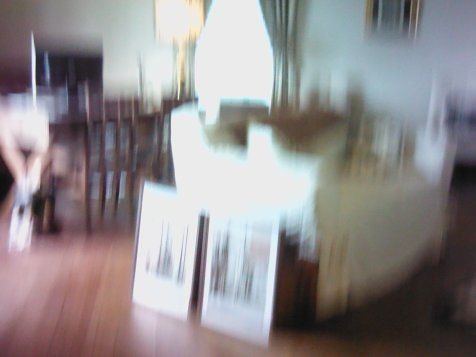This indoor photograph, despite its poor quality and blur, captures a well-lit dining room. The image appears to have been taken in haste, resulting in a lack of focus and clarity. Dominated by a white wall adorned with beige curtains over a window, the setting offers a glimpse of a gold-framed portrait whose details are indiscernible due to the blurriness. In the upper left corner, there is a wooden dining set. The room features elegant hardwood flooring. Central to the image is a white couch, against which two white-framed paintings are propped up.